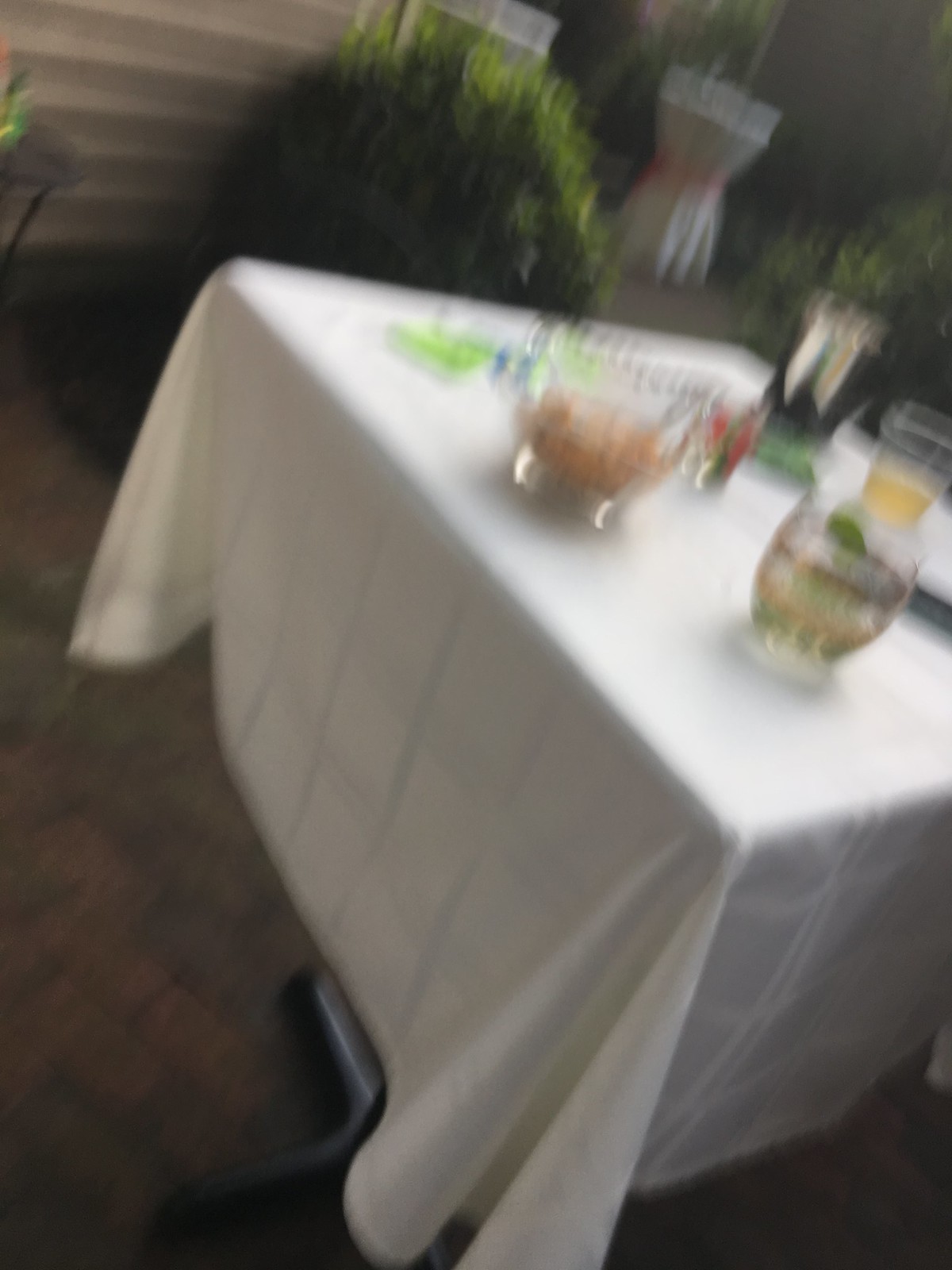A very blurry photograph captures an outdoor setting. The ground is paved with brick flooring, and part of a building can be seen in the top left-hand corner. To the right, a lush green bush adds a splash of color. In the background on the right, there are several tall, high-top tables draped in white tablecloths. Due to the blurriness of the image, the items on these tables are indistinguishable. In the foreground, a regular table also covered with a white tablecloth is visible, adorned with food bowls and drinks. The overall scene is indistinct, making it difficult to discern further details.